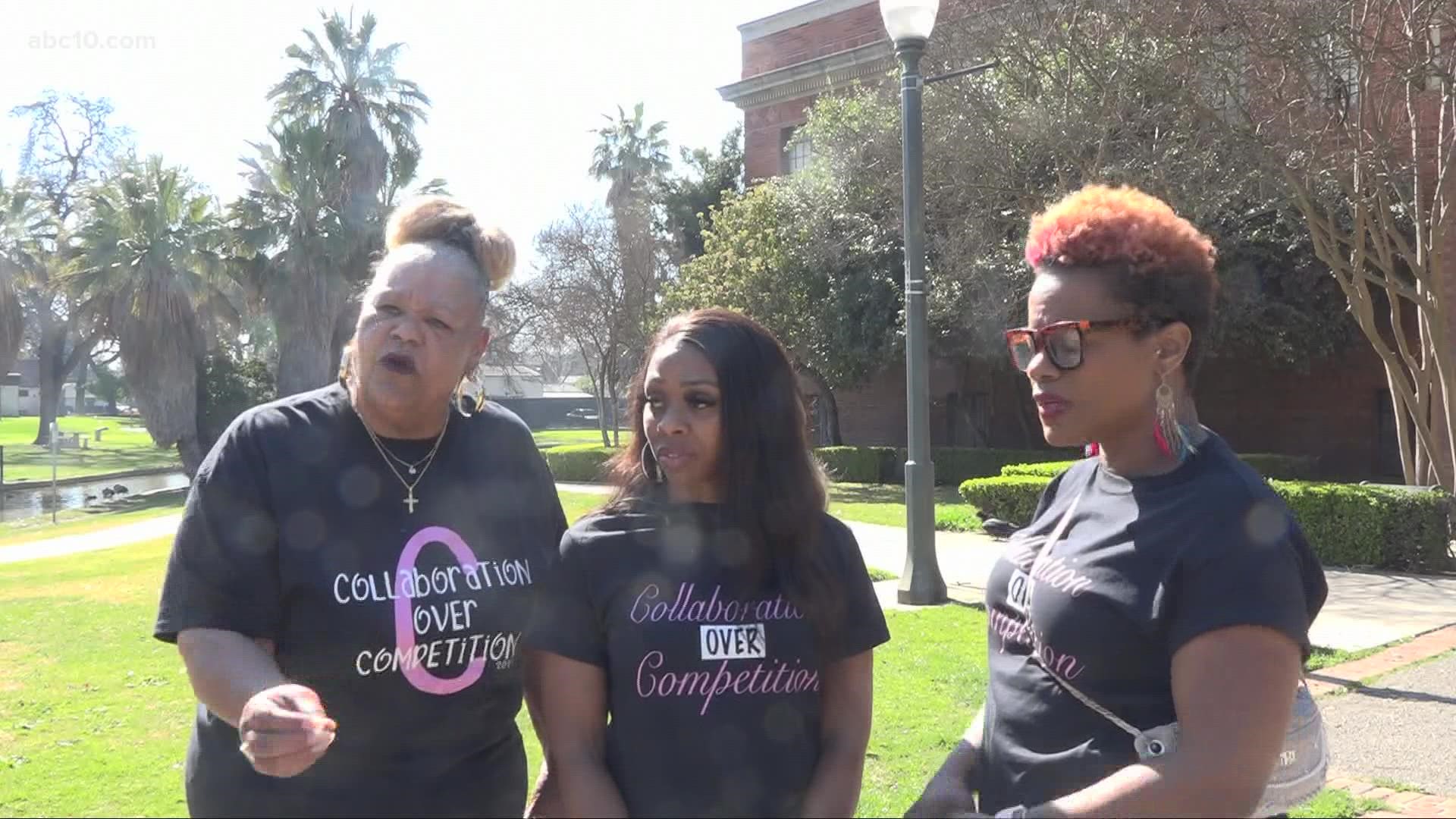This photograph captures three Black women standing outdoors, waist up, under bright daylight. They appear to be in their 40s or 50s and are all wearing black T-shirts with the inscription "collaboration over competition." The woman on the far left is adorned with a gold cross necklace and large gold hoop earrings, her hair styled in a bun, and she wears dark lipstick. Her shirt features the words "collaboration over competition" in white with a prominent purple "C" on the chest. The middle woman, who is shorter with long, straight dark hair, wears a shirt where "collaboration" and "competition" are written in cursive pink, with "over" placed in a white rectangle. The woman on the right, standing sideways, has short, bushy hair dyed red or orange, and wears glasses along with earrings, holding a purse under her arm. She is wearing a similar T-shirt to the first woman. The trio is positioned on a grassy area with a light pole, several palm trees, and a large building, possibly red-bricked, visible in the background. The setting suggests a public or community space, adding to the communal spirit of their attire.